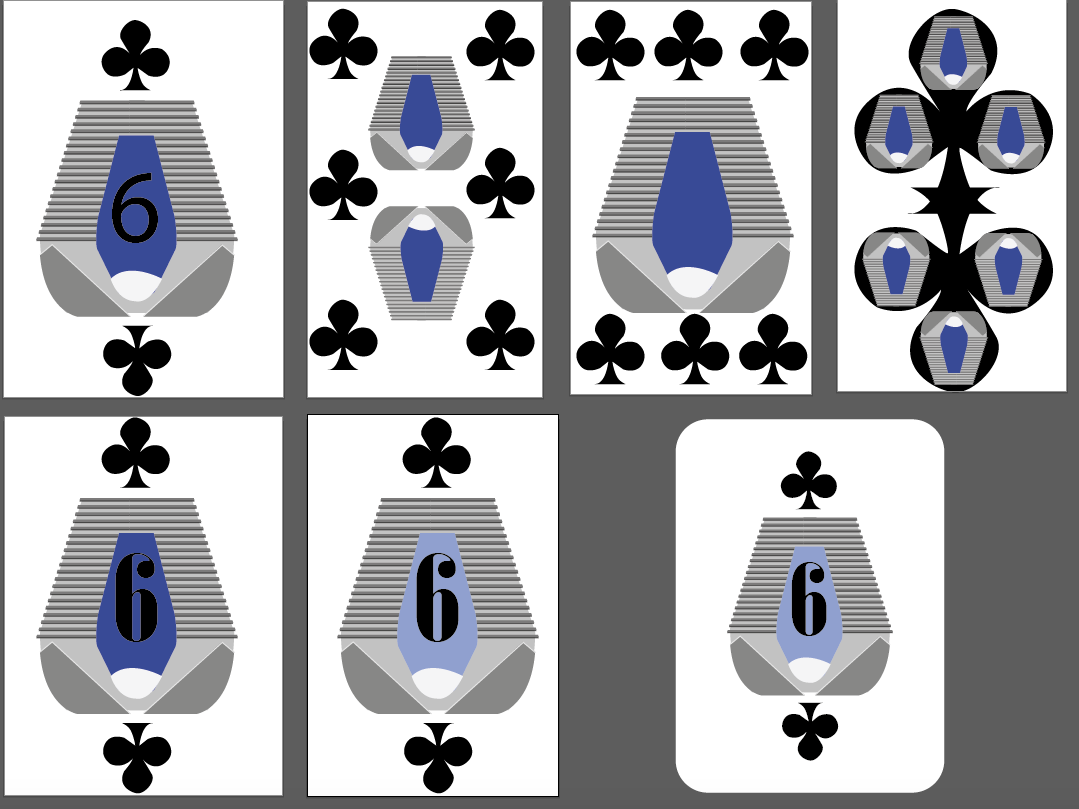The image showcases a collection of seven cards arranged in two rows. The top row comprises four cards, while the bottom row has three cards, with two on the left and one on the right, separated by a space. The cards are predominantly designed with clover symbols and feature recurring geometric patterns. Here’s a detailed description of each card:

1. **First Card (Top Left):**
   - Displays clover symbols on the top.
   - The central area features a distinctive shape resembling a four-sided figure atop a rounded rectangle.
   - At the base center, there's a design similar to a small blue pinkie finger with the number '6' inscribed inside, accented with a hint of white at the bottom.

2. **Second Card:**
   - Contains two identical four-sided shapes, with one oriented upwards and the other reversed.
   - Six clover symbols are present, three on the left and three on the right.

3. **Third Card:**
   - Includes three clover symbols arranged horizontally from left to right at the top and middle sections.
   - A recurring geometric shape with blue filling is located in the center.

4. **Fourth Card (Last in the Top Row):**
   - Features a large clover symbol at the top connected to another clover at the bottom in an inverted 180-degree orientation.
   - Each leaf of the clover contains the familiar grey figure with blue filling.

5. **Fifth Card (Bottom Left):**
   - Exhibits a darker blue geometric central shape with a bolder '6' inside.
   - Highlights a clover symbol at both the top and bottom, arranged in a 180-degree rotated manner.

6. **Sixth Card:**
   - Contains a light blue central shape.
   - Shows one clover symbol at the top and another at the bottom.

7. **Seventh Card (Bottom Right):**
   - Differentiates itself with rounded edges and corners.
   - Displays a clover symbol at both the top and bottom, a '6' in the middle, and has a light blue color instead of the darker blue seen in other cards.

Each card incorporates a combination of clover symbols and geometric designs, maintaining a cohesive yet varied aesthetic throughout the collection.